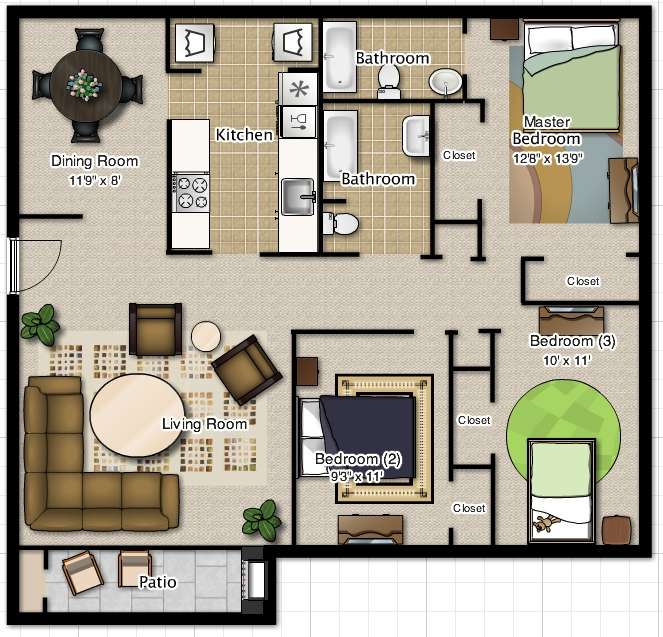This detailed diagram represents an apartment floor plan. The dining room measures 11 feet by 9 feet, adjacent to a compact kitchenette that houses the washer and dryer. Next to the kitchen is the bathroom, equipped with a toilet, tub, and sink. The master bedroom is quite spacious, measuring 12 feet by 13 feet, featuring two closets. 

Below the master bedroom is Bedroom 3, which measures 10 feet by 11 feet and includes one closet. Adjacent to Bedroom 3 is Bedroom 2, measuring 9 feet by 11 feet, and it is furnished with a bed, dresser, and nightstand, all laid out in the floor plan. Bedroom 3 also showcases a twin bed with a table stand and a dresser.

The living room features a sectional couch, a table with two chairs, and two potted plants, creating a cozy gathering space. Across from Bedroom 2, you'll find another bathroom, including a tub, sink, and toilet. 

Additionally, there is a terrace or patio accessible from the main living area, furnished with two chairs. The entryway leads directly into the apartment, integrating seamlessly with the overall layout.